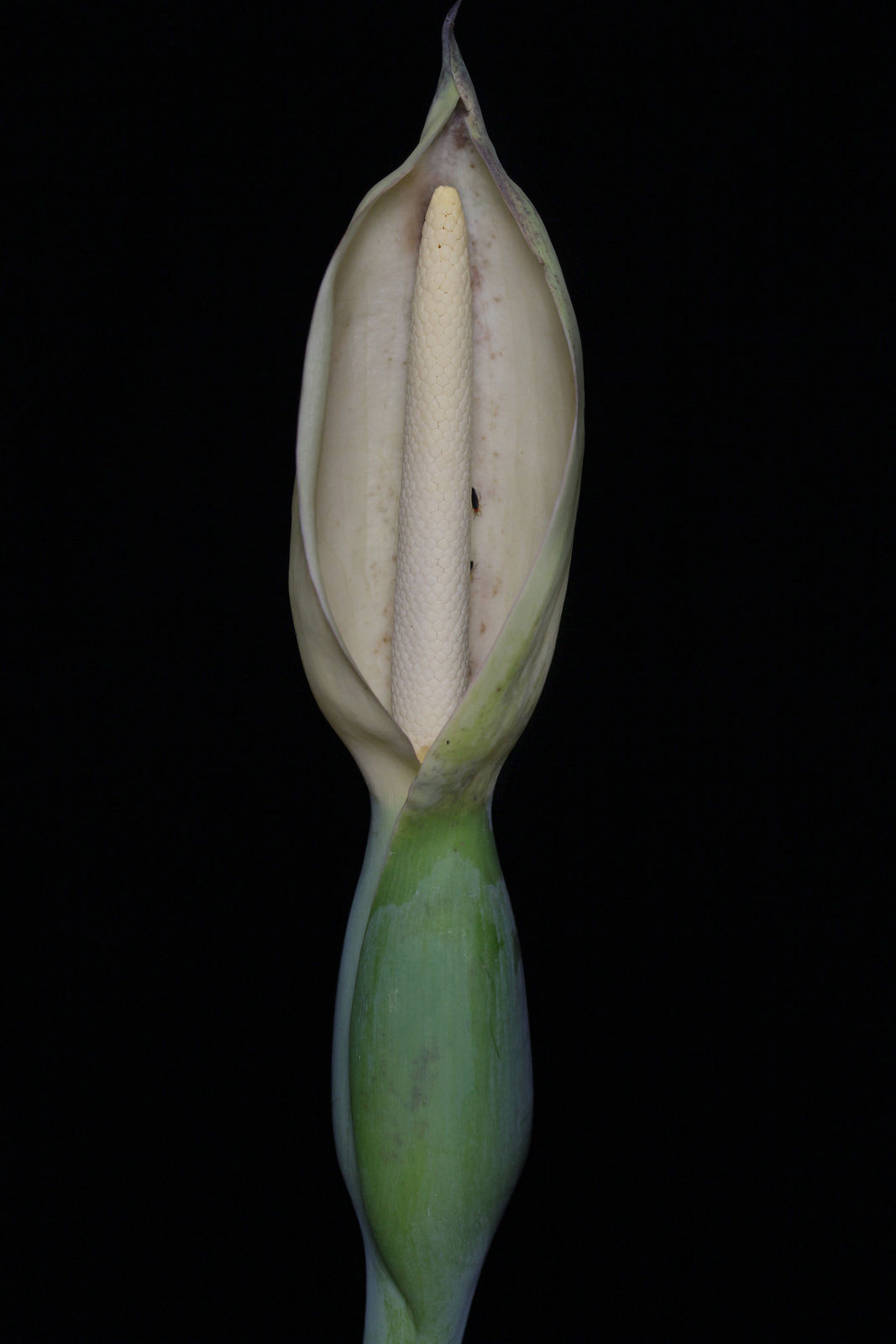This photograph, in portrait orientation, vividly captures a large, tubular seed pod that occupies about a quarter of the image's width, extending vertically from top to bottom. The seed pod, primarily cream-colored with a bumpy texture, is open at the top, revealing its intricate inner structure. Behind this tubular centerpiece, a white cotton-like surface is visible, accentuated by a few small black spots. The exterior of the seed pod consists of overlapping green leaves that taper into a pointed shape at the top and meet at the base, with a hint of blue peeking through the background near the bottom. The entire composition is set against a stark, solid jet-black background, emphasizing the bright and vivid colors of the seed pod and creating a dramatic contrast that highlights the detailed realism of the photograph.